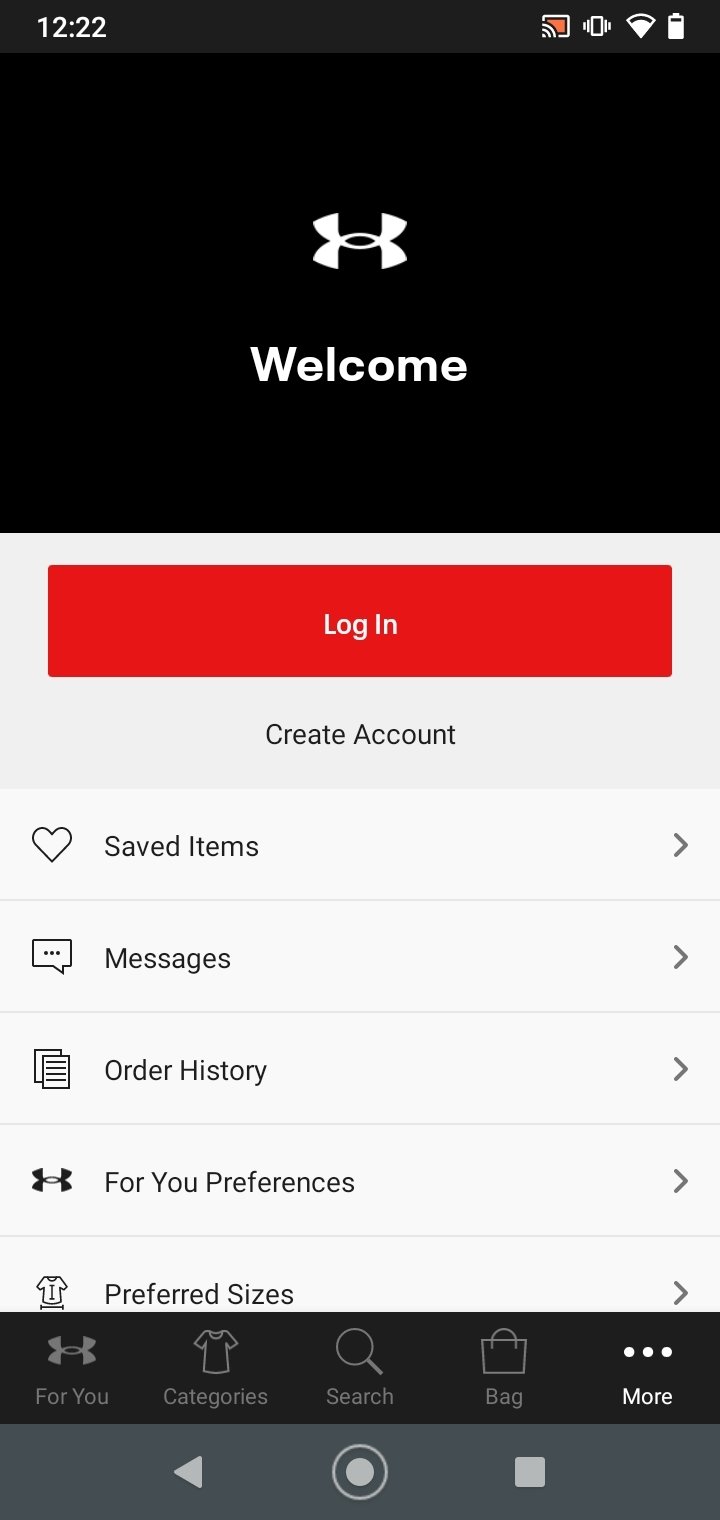The screenshot is of a mobile device, vertically oriented, displaying the Under Armour app. At the top of the screen, there is a prominent black rectangle featuring the Under Armour logo in the center. Beneath the logo, the word "Welcome" is displayed. Below this black section, the screen transitions into the main interface area, which has a clean gray and white design.

In this main section, the first notable element is a horizontal button labeled "Login." Directly underneath this button, there is an option to "Create Account." Below these options, there is a list of menu items, each accompanied by an icon and a right-arrow indicating further navigation. 

- The first menu item is signified by a heart icon and is labeled "Saved Items."
- The second menu item features a message bubble icon and is labeled "Messages."
- The third menu item displays an icon with two pieces of paper, denoted as "Order History."
- Following that is a menu item with the Under Armour logo again, titled "Your Preferences."
- The final menu item shows an icon of a shirt, labeled "Preferred Sizes."

At the bottom of the screen, there is a navigation bar that includes:
- An Under Armour logo with the text "For You."
- A shirt icon with the text "Categories."
- A search icon with the label "Search."
- A bag icon for "Cart."
- An icon with three dots for the "More" options menu.

At the very bottom, the standard phone interface buttons (typically home, back, and recent apps buttons) are visible.